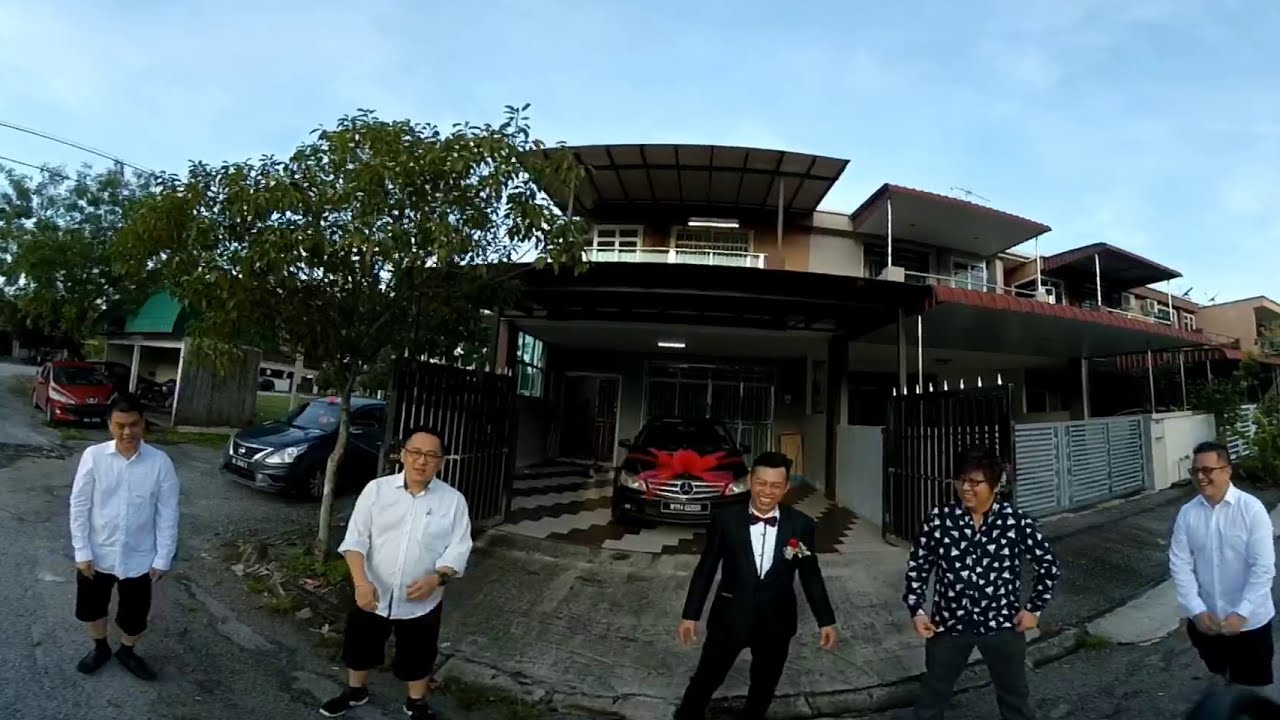In front of a modern, two-story house with blocky design elements, a group of five Asian men pose for a photo on a concrete pavement. Four of the men are casually dressed, with two in white button-down shirts and black shorts—one in black sandals, the other in black shoes and socks. Another man wears a black and white button-down with gray pants and glasses, while the fifth man, also in glasses and black shorts, stands at the far right. The centerpiece of the group is a man in an all-black tuxedo with a white undershirt, a black bowtie, and a red rose in his pocket, suggesting a special occasion. Behind them, a black Mercedes adorned with a red ribbon sits in the driveway, indicating it might be a gift for the tuxedoed man. Flanking the Mercedes are a blue car and a red car, with additional housing structures visible in the background. The area showcases green trees, green grass, and a striped black-and-white or gold-and-white floor pattern. Overhead, a blue sky with thin white clouds completes the scene. The image, apparently taken with a wide-angle action camera, captures the celebratory atmosphere and detailed surroundings.